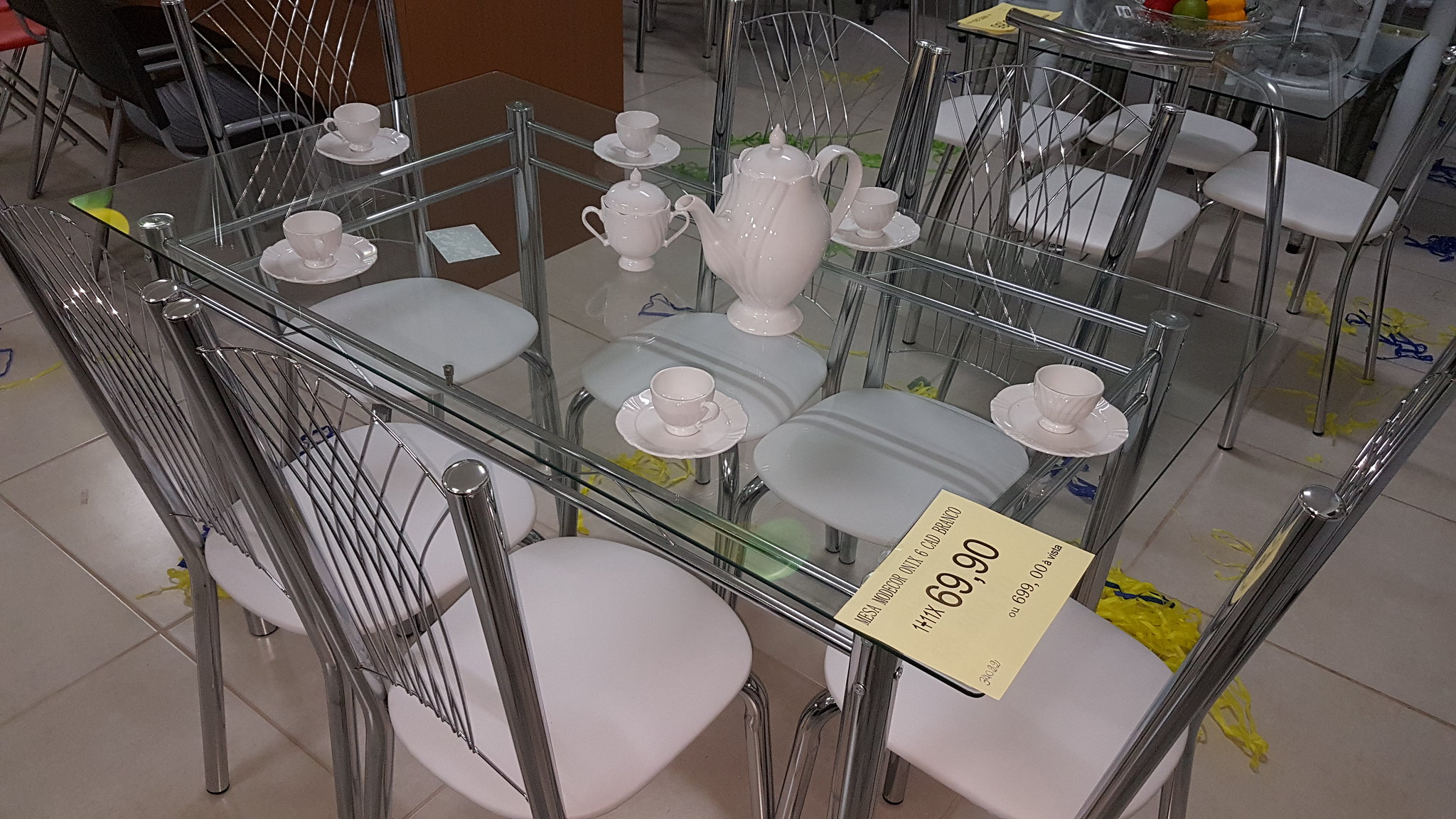The photograph captures a minimalistic chrome and glass dining table set prominently displayed in what appears to be a showroom, likely a second-hand or furniture store. The table features a clear glass rectangular top supported by sleek chrome metal legs. Arranged around the table are six matching chairs, each with a white seat cushion and a chrome back adorned with art deco-inspired arched wire designs. In the center of the table, a white tea set consisting of a teapot, a sugar container, and six cups with saucers is laid out, creating an elegant and inviting scene. A price tag on the table reads $69.90, although the exact currency is uncertain. The setting is accented by large grey and white tiled flooring, and other similar dining sets are visible in the background, reinforcing the showroom ambiance. The overall lighting of the photo is somewhat dim, adding to the cozy atmosphere of the display.